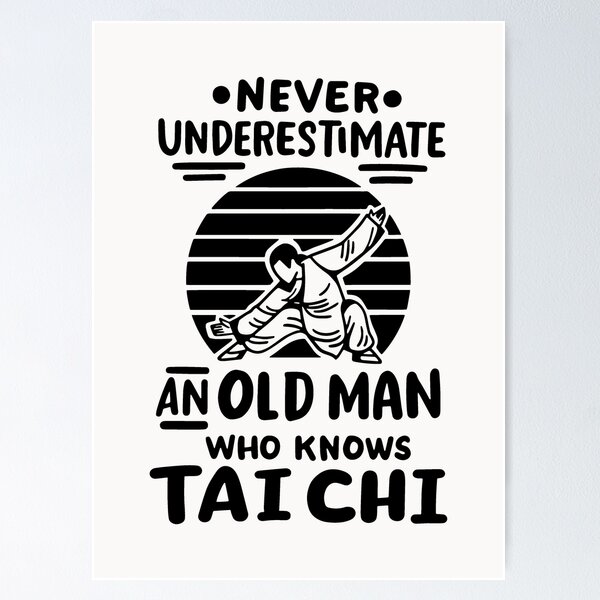This is a monochromatic poster set against a light gray background featuring a black and white design on a white surface. Dominating the center is a black circle resembling a sunburst, segmented into several rectangular shapes, evoking the iconic rising sun imagery. In front of this sun, a simplistically drawn man in a Tai Chi pose is depicted in black outline, crouched forward on one knee with his arms at an angle and eyes looking downwards. He is dressed in flowing robes, and his form lacks detailed facial features, emphasizing his silhouette. Above this central image, the poster reads in black text, "Never • Underestimate •", with double underlines separating "und" and "mit" in "Underestimate." Below the sunburst and figure, it states, "an old man who knows Tai Chi." The overall style is a primitive black and white illustration, giving it a timeless, almost zen-like quality appropriate for various settings, especially a gym.